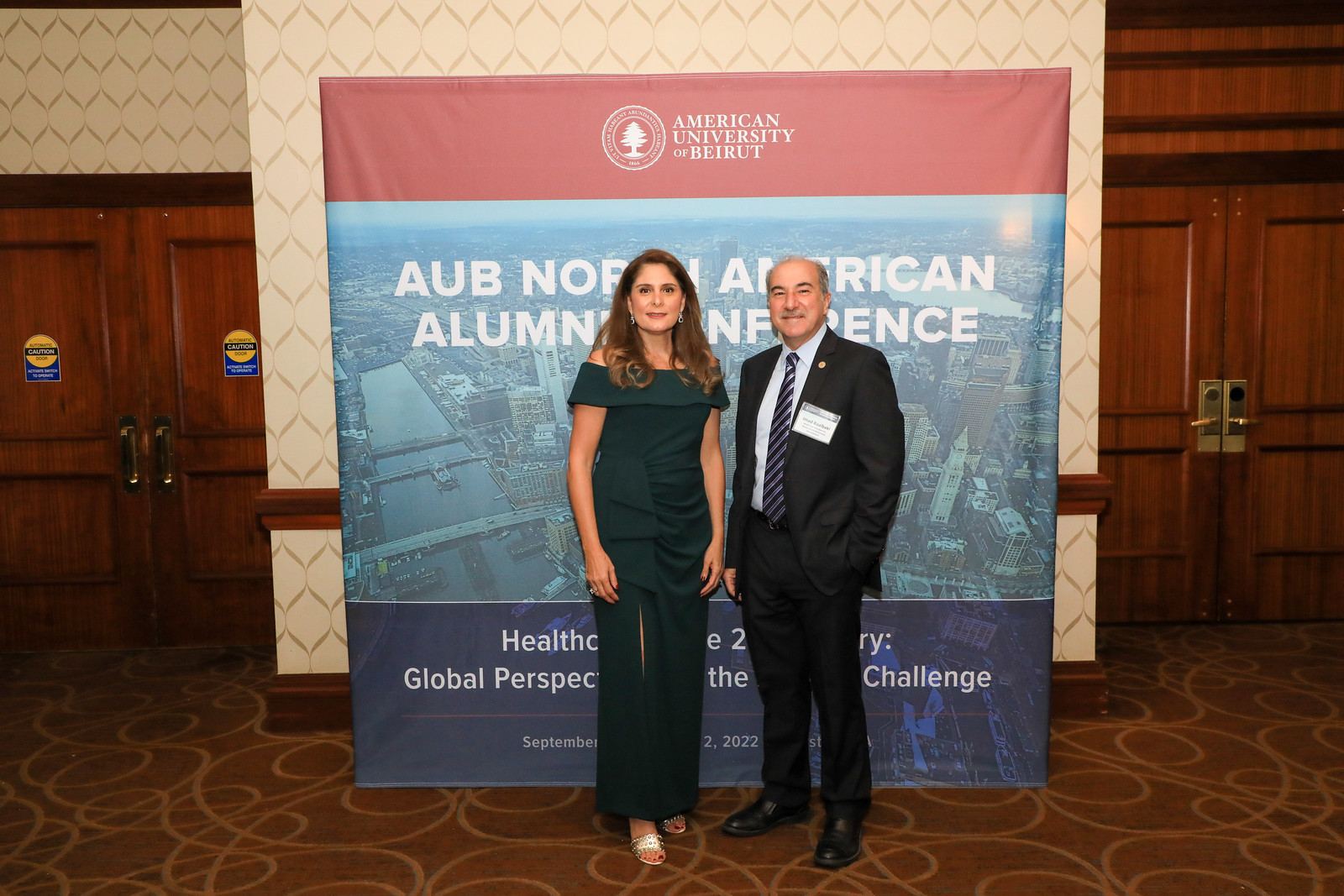The photograph, taken indoors and rectangular in shape, captures two individuals standing in front of a large banner on a yellow wall. The image is wider than it is tall. The floor is covered in a brown carpet featuring light golden swirl designs. On each side of the wall, wooden double doors, currently closed, are visible.

In the image, a man and a woman are positioned slightly left of center. The woman, who is Caucasian with long brown hair curled at the shoulders and parted on the side, is wearing a green off-the-shoulder gown with a slit on the right leg and silver open-toed dress shoes. She is standing on the left and looking directly at the camera, accessorized with earrings.

The man, also Caucasian, has balding hair with gray over the temples and a mustache. He is dressed in a black dress jacket, slacks, a blue collared button-up shirt, and a blue and gray striped tie. A pin adorns the lapel of his jacket.

Behind them, the banner features a red header with a white circle containing a tree logo. To the right, it reads "American University of Beirut." The lower section of the banner has a blue background with an image of a city and white print, displaying the letters "AUB," followed by partially obscured words that may include "American," "alumni," "conference," "health," "global perspective," "challenge," and the date "September 2022."